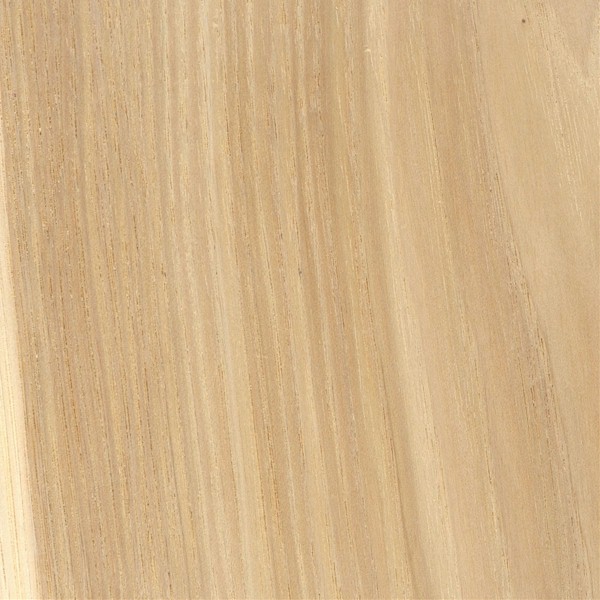This extreme close-up image showcases a simple yet detailed wood grain pattern, likely from a plank of wood, possibly used for flooring or a tabletop. The grains run in long, vertical stripes with multiple shades of brown, predominantly light brown. There's a noticeable blonde strip on the far left, transitioning into slightly darker tones and then back to lighter hues. The wood appears raw and unfinished, suggesting it might be freshly cut or sanded and prepped for varnishing or painting. The surface is smooth, indicating a recent sanding. There are occasional darker patches and small black specks visible, adding to the textural detail of the wood. Overall, the image captures the natural and varied beauty of a light-colored, unvarnished wooden surface.